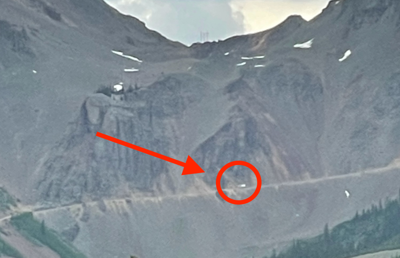This image captures a blurry, aerial view of a steep mountain range with a treacherous winding road carved into its side. The foreground of the photo shows sparse greenery and scattered trees, while the majority of the mountain is gray and rocky, with exposed cliffs and occasional patches of snow. Dominating the scene is a large red arrow pointing to a circled area on the road, which highlights a vehicle navigating this precarious route. The road appears dangerously close to the edge, underscoring the perilous nature of the descent. The background includes a small expanse of sky with clouds, adding to the expansive feel of the landscape.